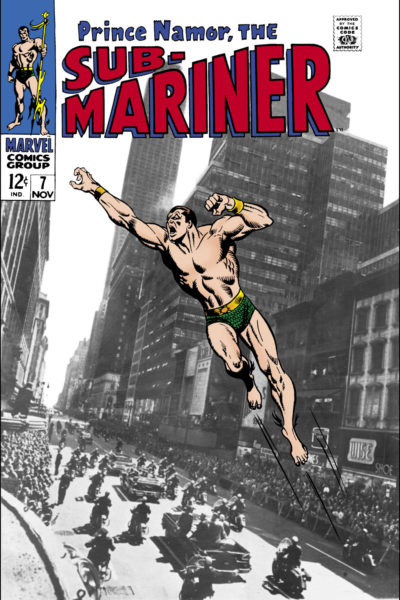The comic book cover depicts "Prince Namor, the Submariner," a Marvel superhero. The background features a black-and-white photograph of John F. Kennedy's motorcade, with black cars and motorcycles proceeding down a crowded street lined by tall buildings, echoing a 1960s parade scene. Superimposed on this historical backdrop is a colorful illustration of Prince Namor. He is heroically posed, seemingly flying or jumping through the air. Namor is muscular, with a bare chest, and wears distinctive green trunks, gold wrist bracelets, and a gold bangle on his upper left arm. The title "Prince Namor" is in blue, while "the Submariner" is prominently displayed in large red block letters. In the upper left corner, "Marvel Comics Group" is printed in navy blue along with "12 cents" and "November 7th" in black, giving it an authentic vintage comic book feel.